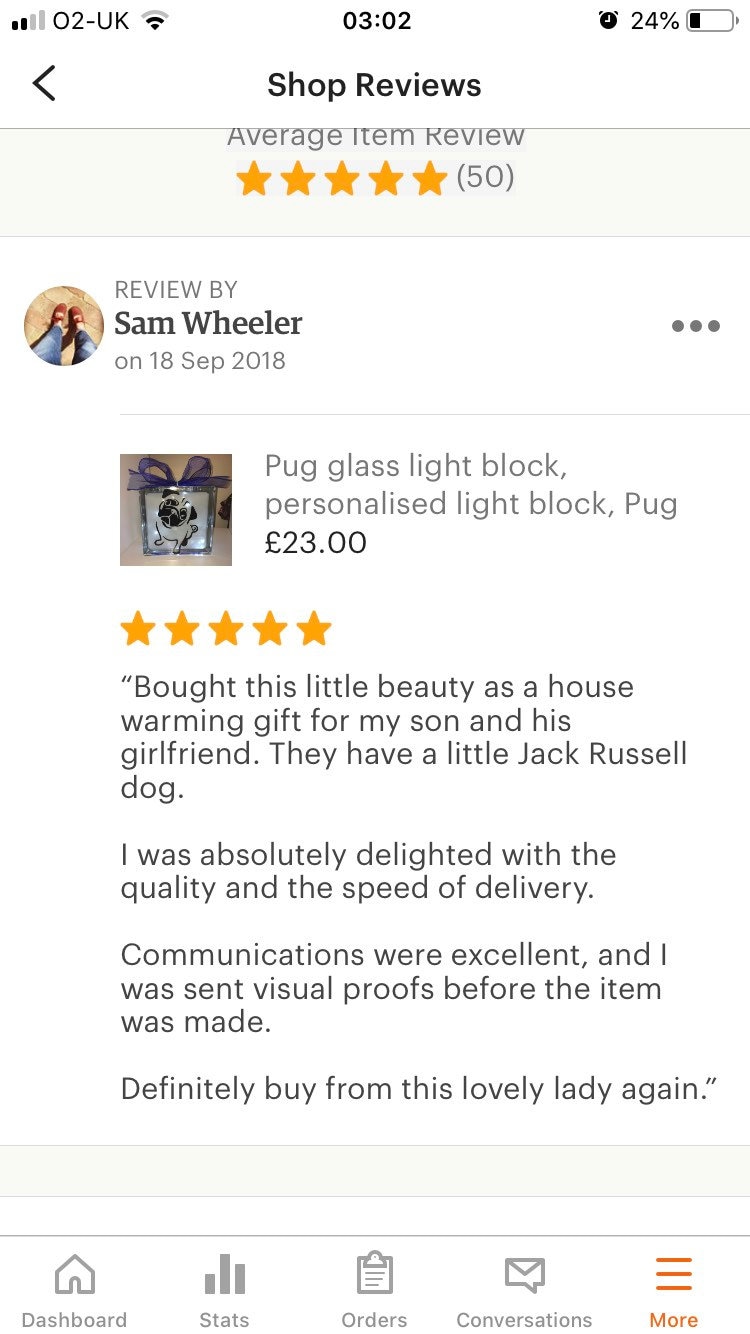Screenshot of a Product Review 

At the top of the image, it is labeled "Shop Reviews." The main content shows a review left by Sam Wheeler in September 2018 for a "Pug Glass Light Box," a personalized light block priced at 23 euros. The review has a 5-star rating. In the review text, Sam Wheeler states: "Bought this little beauty as a housewarming gift for my son and his girlfriend. They have a little Jack Russell dog. I was absolutely delighted with the quality and speed of delivery. Communications were excellent, and I was sent visual proofs before the item was made. Definitely buy from this lovely lady again."

Below the review, the interface lists options such as Dashboard, Stats, Orders, Conversations, and more. The top section also mentions that the average item rating is 5 stars across 50 reviews. A small image of the product—a glass box with a purple ribbon, featuring a photo of a dog—is included. The background of the review is white, and the text is black.